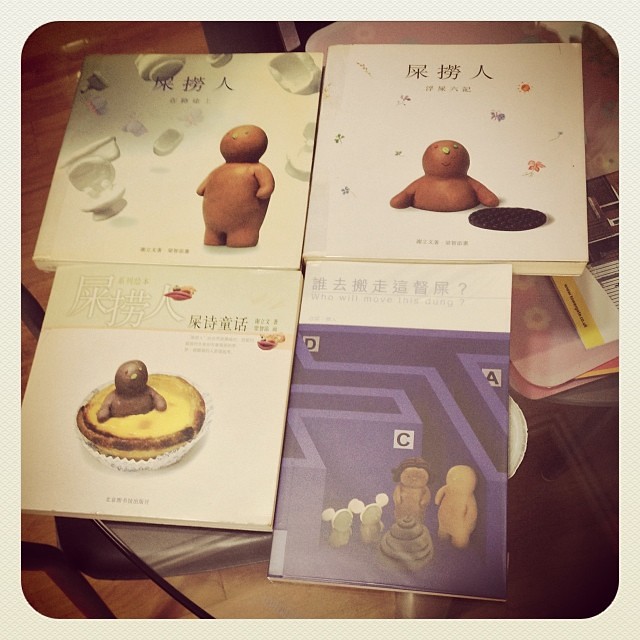The photograph depicts four books laid out on a glass table, with each book displaying a unique illustration of a small, brown, clay figurine that closely resembles the Pillsbury Doughboy but with no clothing. The book titles are all written in either Japanese or Chinese characters.

1. **Top Left Book**: This book features a green cover with the clay figurine standing and looking off into the distance. In the bottom right corner, there is a white book decorated with small flowers.
   
2. **Top Right Book**: The clay figurine appears partially submerged, like he's stuck in a manhole, with only his upper half visible. A small, round, black object resembling an Oreo cookie is positioned near him, amidst various white decorative pieces.

3. **Bottom Left Book**: The figurine is seen emerging from what appears to be a custard pie, complete with a white pie holder and a yellow and green background. This backdrop extends to about three-quarters of the image.

4. **Bottom Right Book**: This book displays two clay figurines standing beside one another. One has hair, and the other is bald. Accompanying them are two smaller, mouse-like figures, and the book itself has a maze design. Distinct letters "C," "D," and "A" are visible within the maze, and two smaller gray figures with round ears are also present.

The detailed illustrations and the use of vibrant colors are consistent across all books, making the figurines the central theme. This suggests that the books could be part of a series, possibly calendars or storybooks. The books rest on a table adorned with a placemat or cloth, adding to the still-life composition.